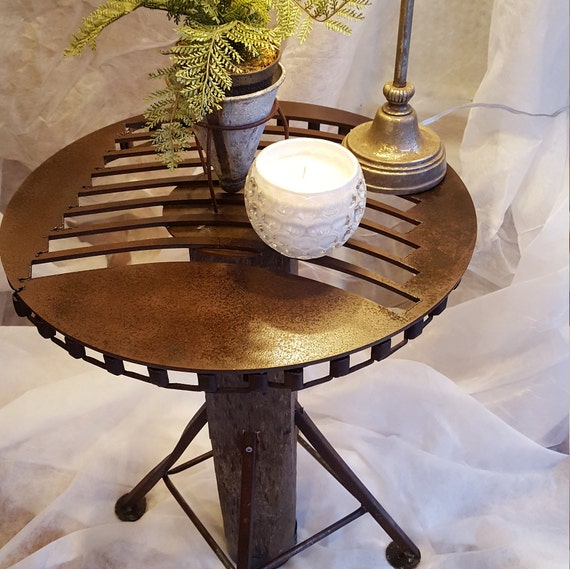The image depicts a small, round metallic table with a wooden base featuring three visible legs. The tabletop is designed with a series of curved, rainbow-shaped slits that create a unique pattern. The table is set upon a crumpled, white fabric that resembles a linen or sheer curtain, which extends into the background. On the surface of the table sits a white candle votive, slightly off-center to the right, a conical metallic planter with a green fern, and the base of a metallic lamp with a white electrical cord trailing off. The table, planter, and candle holder's arrangements suggest an indoor setting, illuminated by a light source from above.